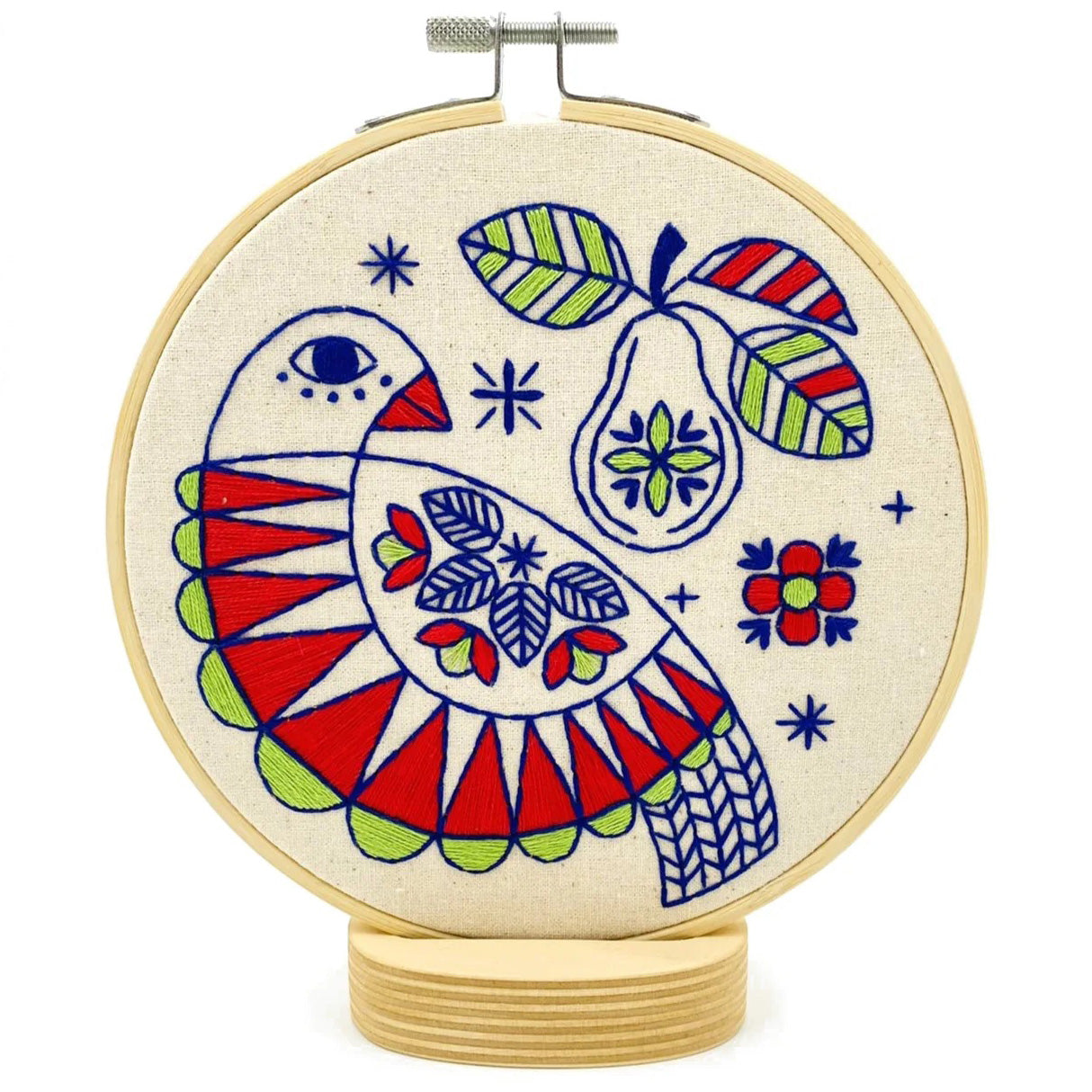The image showcases an intricate cross-stitch design set within a circular, light brown wooden frame, commonly used for embroidery. The frame is approximately four inches wide and five inches tall, complete with a tightening screw at the top for adjusting tension. This frame sits on a light brown wooden base, roughly one inch high and an inch and a half to two inches wide, providing stable support.

The background of the cross-stitch pattern is a light tan, fabric-like canvas. On the bottom left of the design, there's a detailed depiction of a bird. The bird features a body oriented towards the left but appears to be glancing over its shoulder to the right. Its eye is blue, and it has an orange beak. The bird's body is adorned with alternating triangles of white and red threads, a green patch under its belly, and a white wing decorated with blue leaves and red and green flowers.

Adjacent to the bird, in the upper portion of the pattern, is a pear. The pear is characterized by stripes in various colors. Three leaves sprout from it—two exhibiting green and white stripes, and one with orange and white stripes. Additional smaller elements, such as red flowers and blue leaves, are scattered around the primary motifs, enhancing the vibrancy of the piece.

Overall, the design is a harmonious blend of blue, red, green, and white threads against the beige canvas, framed elegantly within the wooden perimeter, making for a captivating and colorful art piece.